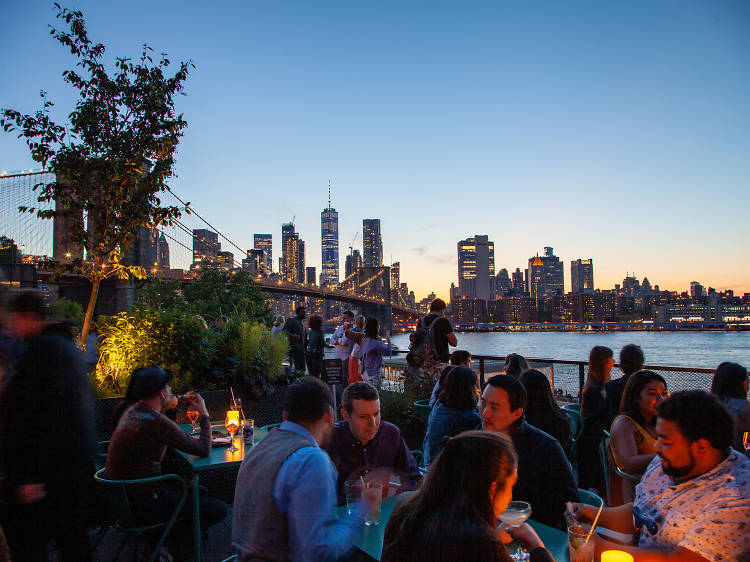This detailed photograph captures the lively ambiance of an outdoor bar situated on a dock next to a serene body of water, likely a river or bay. The setting sun bathes the scene in soft hues of yellow, peach, and blue, signaling the onset of dusk. The backdrop boasts a stunning cityscape of New York City, with twinkling lights beginning to illuminate the skyline. Dominating the background, a large bridge, likely the Brooklyn Bridge, stretches from the far left to the center of the image. In the foreground, a diverse crowd of people of various races, genders, and ages sit around candlelit tables, enjoying alcoholic drinks and possibly small appetizers. The air seems filled with the buzz of conversation and shared stories. Light attire and blooming trees hint at a pleasant spring or summer evening. The overall atmosphere exudes a sense of comfort and camaraderie as friends revel in the picturesque setting.